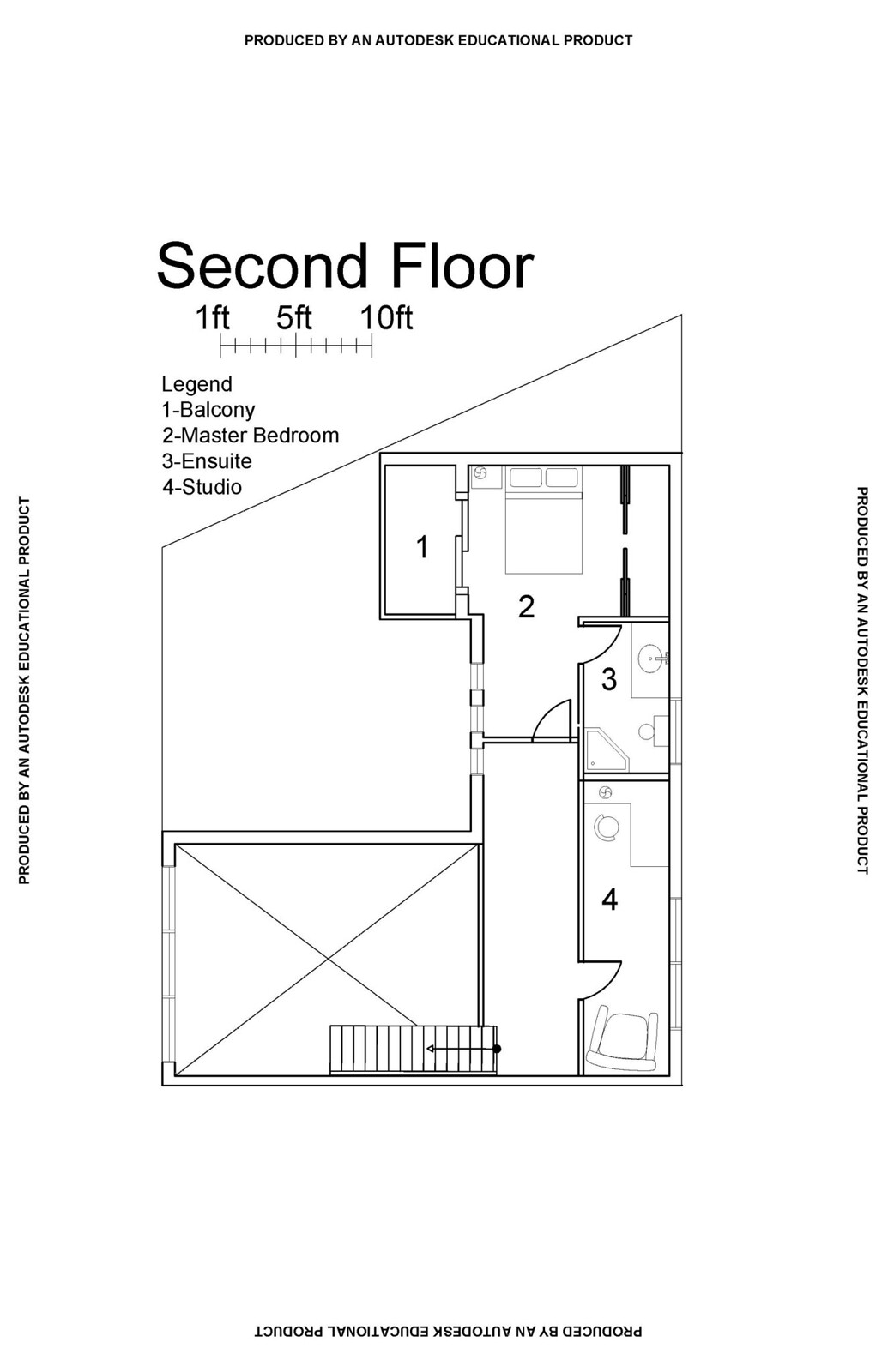This detailed black and white floor plan, created using an AutoCAD-type drawing tool, illustrates the second floor layout. At the top of the vertical image, a caption prominently declares "Second Floor," accompanied by a scale indicating measurements from 1 foot to 10 feet. Adjacent to this is a legend outlining the key areas on the second floor: a balcony, master bedroom, en suite, and studio. Three sides of the diagram are labeled with the note that it was produced by an Autodesk educational product.

The slightly rectangular layout is distinct, with the top edge cut diagonally at approximately a 45-degree angle. The diagram features stairs located at the bottom center, leading to a hallway or balcony area. This corridor provides access to a separate studio entrance. At the end of this hallway, a door leads into the spacious master bedroom, with an en suite bathroom conveniently situated just inside the door to the right. The master bedroom boasts sliding glass doors that open directly onto the balcony, offering an extension of the living space outdoors.